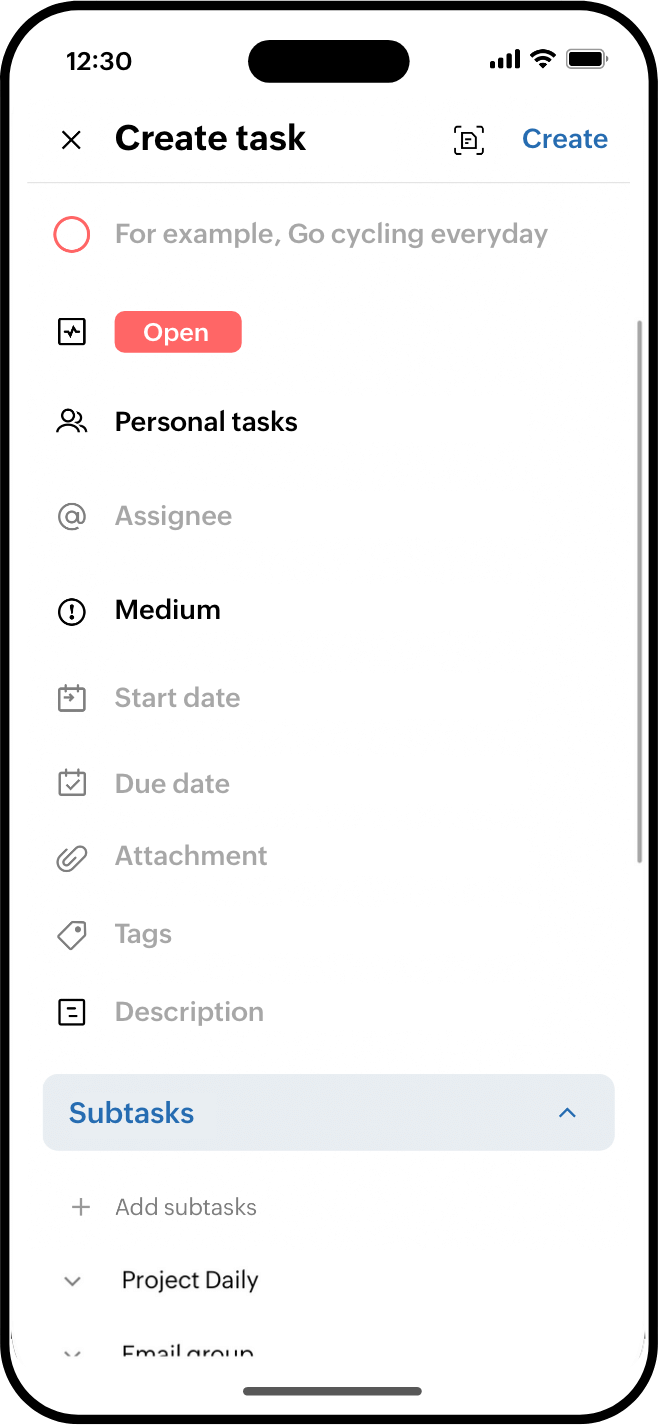A screenshot of an iPhone, possibly an iPhone 14 or 15, appears on a white background. The image resembles an emulator screen or a digitally drawn boundary, showcasing the black island at the top of the iPhone's display. The status bar shows the time as 12:30 with four bars of cellular reception, full Wi-Fi signal, and a fully charged battery, all depicted in black icons. At the bottom of the screen, the home bar is visible. 

The primary focus of the screenshot is an app interface, most likely a task management or exercise app, also set against a white background. Towards the bottom, there is a blue-text heading labeled "Subtasks" with a light blue background, and an arrow icon indicating the option to expand the menu. Above this, there's a section labeled "Create Tasks" with a red-circle icon. This section includes placeholder text in grey, such as "Go Cycling Every Day," and a red "Open" button. Other options like "Personal Tasks" and "Medium" are in black text, while fields like "Assignee," "Start Date," "Due Date," "Attachment," "Tags," and "Description" are all greyed out, suggesting they are inactive or unfilled.